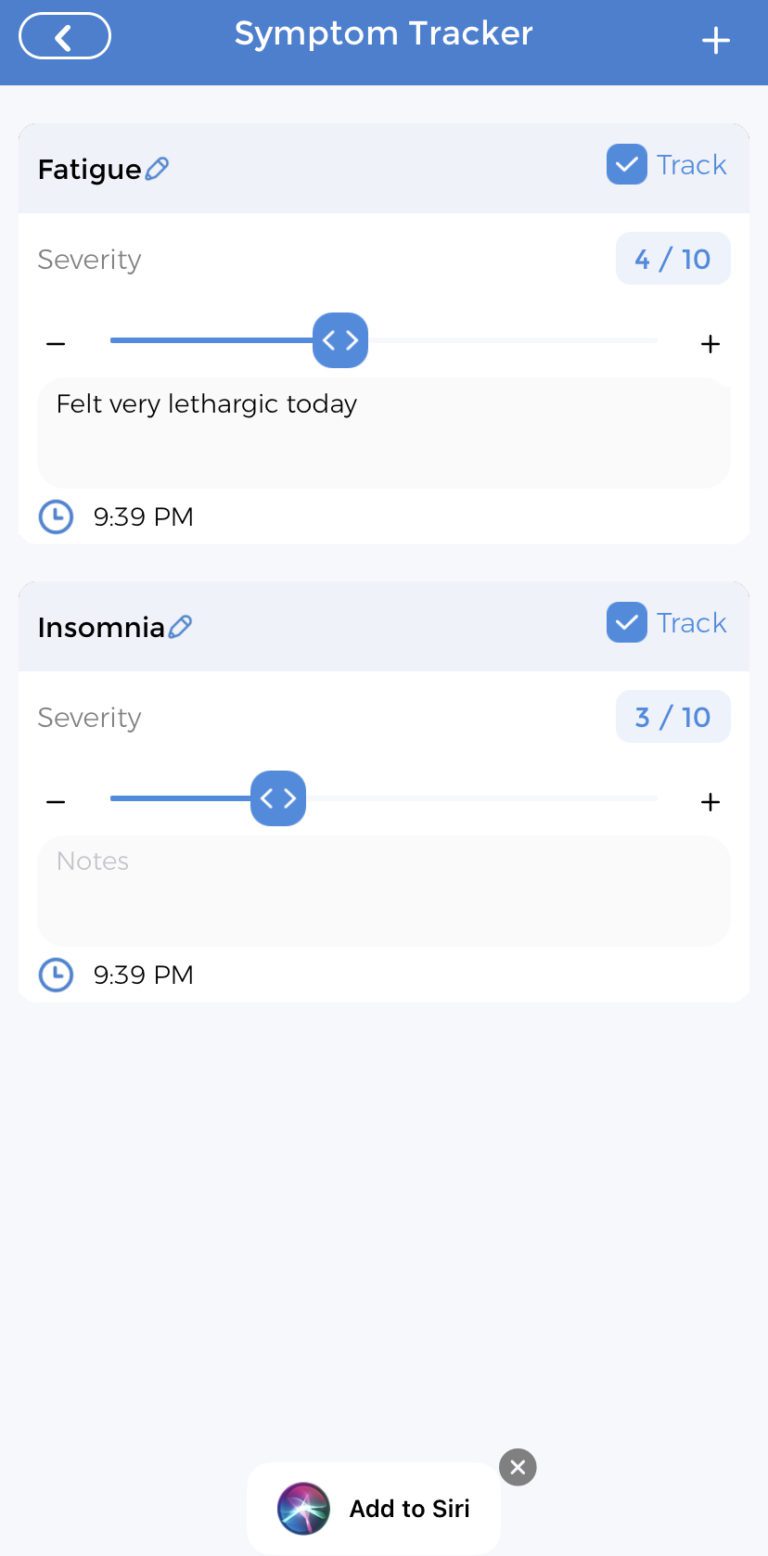This screenshot is taken from a health app, specifically showcasing the symptom tracker panel. At the top, the title "Symptom Tracker" is centered within a blue header bar. On the far left of this header, a left-pointing arrow is enclosed within a white-outlined oval, indicating a back option, while a plus sign on the far right allows the user to add new information.

Directly below the blue header, a box labeled "Fatigue" appears in the top left, next to a blue pencil icon that allows editing of the title. Adjacent to "Fatigue" is a checked checkbox labeled "Track," signifying that fatigue tracking is active. Underneath, a white box labeled "Severity" contains a slider bar set at 4 out of 10. Below the slider, there is a note stating, "Felt very lethargic today," time-stamped at 9:39 PM with a clock icon on the bottom left of the note.

Further down, the screenshot includes a section for tracking insomnia, with a similar format. "Insomnia" is written on the left, with a pencil icon next to it for editing, followed by a checked checkbox labeled "Track." A white box labeled "Severity" shows a slider set to 3 out of 10. Unlike the fatigue section, this one contains no additional notes, only a placeholder text in light gray stating "Notes." This section is also time-stamped at 9:39 PM, indicated by a clock icon on the bottom left.

At the very bottom center of the screenshot, there is an "Add to Siri" option, with an 'X' on the top right corner of the panel, likely to dismiss the Siri addition prompt.